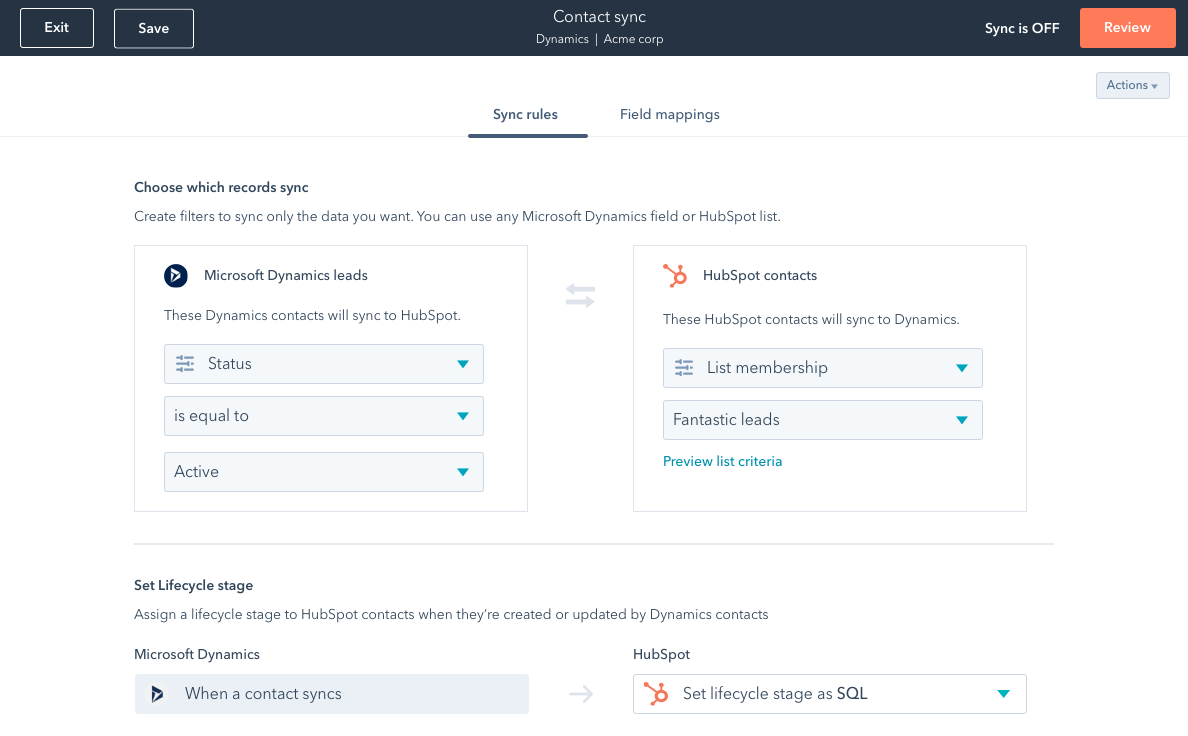The image depicts a settings page on a website, specifically dedicated to contact synchronization between Microsoft Dynamics and HubSpot, under the banner "Contact Sync, Dynamics, Acme Core." At the top left, there are two buttons: an exit button and a save button. To the top right, there is a note indicating "Sync is off," accompanied by an orange "Review" button, all positioned on a black horizontal bar.

Below this bar, two tabs are visible: "Sync Rules" and "Field Mappings," with "Sync Rules" currently selected. The instructions under the "Sync Rules" tab state, "Choose which records sync. Create filters to sync only the data you want. You can use any Microsoft Dynamics field or HubSpot list."

The left section is dedicated to "Microsoft Dynamics leads" and details that "These Dynamics contacts will sync to HubSpot," with a filter specified as "Status is equal to Active." 

On the right, the "HubSpot contacts" section explains that "These HubSpot contacts will sync to Dynamics," listing two specific attributes: "List membership with a filter 'Fantastic Leads'."

At the bottom, there is a section for setting the lifecycle stage. Users can assign a lifecycle stage to HubSpot contacts when they are created or updated by Dynamics contacts, with an example showing "When a Dynamics contact syncs, set HubSpot lifecycle stage as SQL."